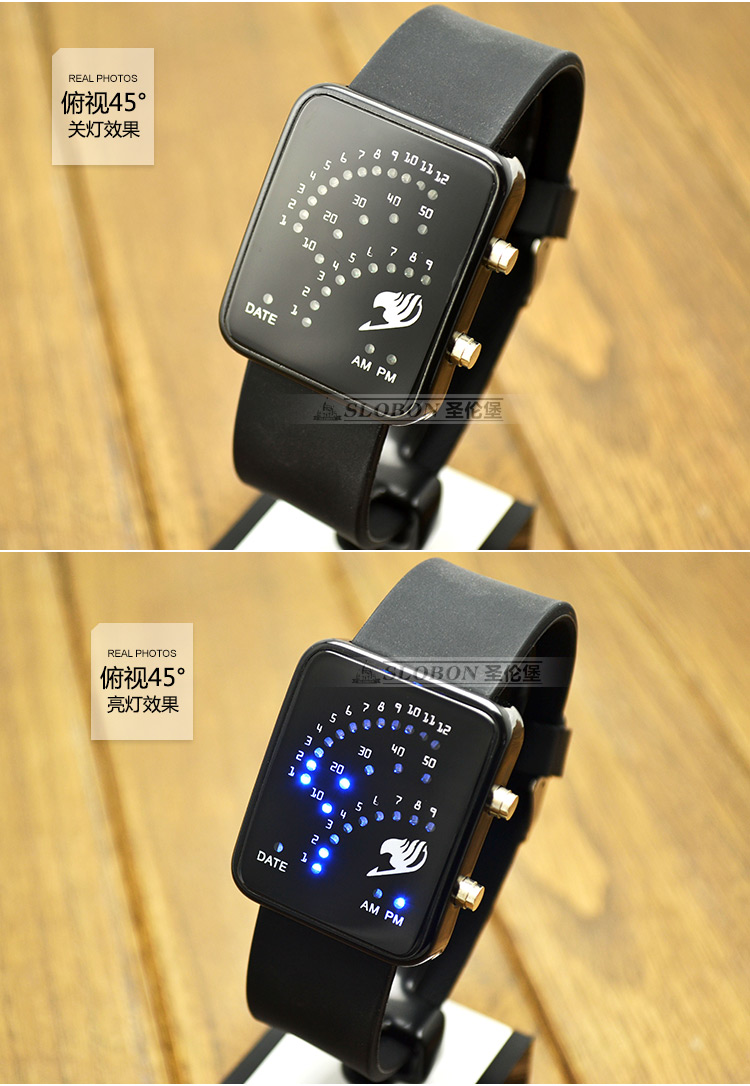This frame features two separate images of the same black watch with a wide, smooth band, displayed one on top of the other against a light brown wooden surface. The watch has a square face with a black background. Within the face, the numbers are laid out in semi-circular arcs: 1 through 12 at the top, 1 through 9 in the middle, and 10, 20, 30, 40, 50 at the bottom. In the top-right corner of the watch face is a small bird logo, and the date, along with AM and PM indicators, are positioned at the bottom-left and bottom-right corners respectively. The notable feature of this watch is the tiny LED lights that illuminate in a light blue to display the time and date; these lights are not illuminated in the top image but are active in the bottom image, showing a practical representation of how the display looks when in use. Both images are bordered by a white frame and a small note in Japanese is visible, reading "real photos" and "45 degrees," although the rest of the text remains unreadable.